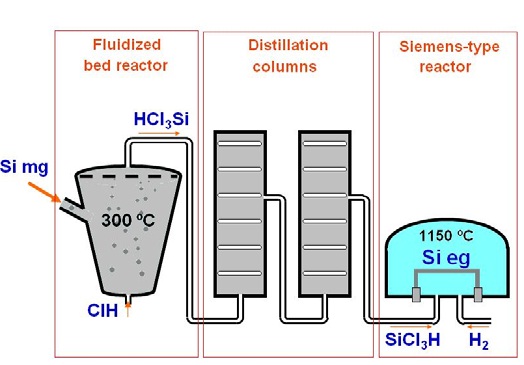The image is a horizontally aligned composite diagram depicting an industrial chemical process, divided into three vertical segments, each with its own title at the top in brown text. 

The first segment on the left illustrates a fluidized bed reactor, represented by a gray tank resembling a cup, marked at 300°C. This section shows an input funnel labeled SIMG with an arrow directing towards it, and beneath the tank, an outlet labeled CIH. Additionally, a hose labeled HCl3Si connects this reactor to the next segment towards the right.

The middle segment features two vertical rectangular containers labeled as distillation columns. These columns are interconnected by several hoses, indicating the movement and separation of chemical substances between the columns.

The rightmost segment displays a Siemens-type reactor characterized by a blue, dome-shaped structure. This reactor operates at 1150°C and involves a chemical reaction denoted by SIEG. Two tubes are connected to this reactor: one labeled SiClH directs input into the reactor, and the other labeled H2 indicates an output.

Overall, the image provides a detailed visual breakdown of a chemical distillation and reaction process across three distinct reactors.